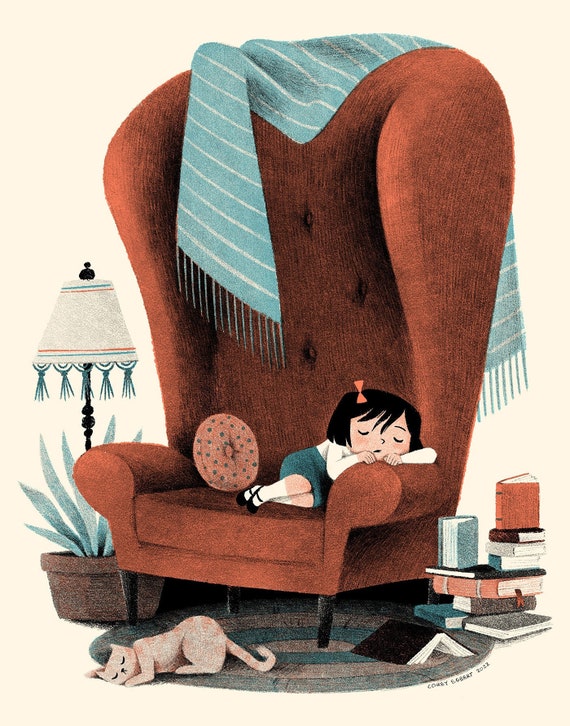In this detailed, vintage-style illustration reminiscent of a mid-century storybook, a large, exaggerated red armchair serves as the focal point. The chair, with its unusual proportions, makes the little girl asleep on its right armrest appear almost cat-sized. She has short black hair adorned with an orange ribbon and is dressed in a white long-sleeve shirt with a dark blue-green skirt, white socks, and black shoes. Resting against the armchair is a blue and white striped shawl and a small circular pillow, orange with blue dots. Below the chair, a grayish-white cat with orange stripes sleeps on a green and gray circular rug. To the left of the armchair, a night lamp stands with a plant beneath it, while to the right, there is a stack of books, suggesting the girl fell asleep while reading. The image captures a nostalgic, tranquil scene, evoking the cozy charm of classic children's book illustrations or vintage magazine covers like those of The New Yorker.